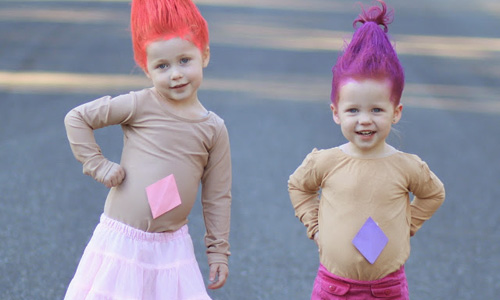In this charming photograph, two young girls are dressed as troll dolls, complete with whimsical, cone-shaped hair that mimics the iconic troll doll look. The girl on the left sports bright orange-pink hair pulled up into a triangular style, while the girl on the right showcases vibrant purple hair styled similarly. Both their hairstyles are secured in a way that makes the hair stand upright, reminiscent of the wild, gelled hair of classic troll dolls.

The girls are wearing skin-toned, long-sleeve shirts to give the illusion of the dolls' rubbery bodies. Adorning their outfits are paper diamonds taped onto their belly buttons, with the left girl's diamond shaded pink and the right girl's diamond shaded purple. Below their shirts, the girl on the left wears a light pink dress, and the girl on the right is in bright pink shorts. They stand on a gray asphalt street, possibly preparing to go trick-or-treating, evoking the joyous spirit of Halloween. The girls' playful costumes and joyful expressions capture the whimsical essence of their cosplay.